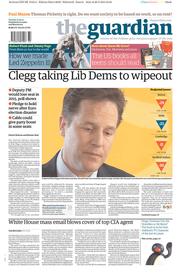In this image, we see a newspaper from The Guardian, though the text is largely illegible due to significant degradation in image quality. A prominently featured headline reads: "Clegg Taking Lou Dames to Wipe Out." The image also captures the distressed visage of a man clad in a suit with a white shirt underneath, conveying a sense of sadness. Another notable headline states: "White House Mass Email Blows Cover of Top CIA Agents." The color palette of the image includes white, blue, red, pink, and orange, adding a varied yet muted visual texture to the newspaper's presentation.